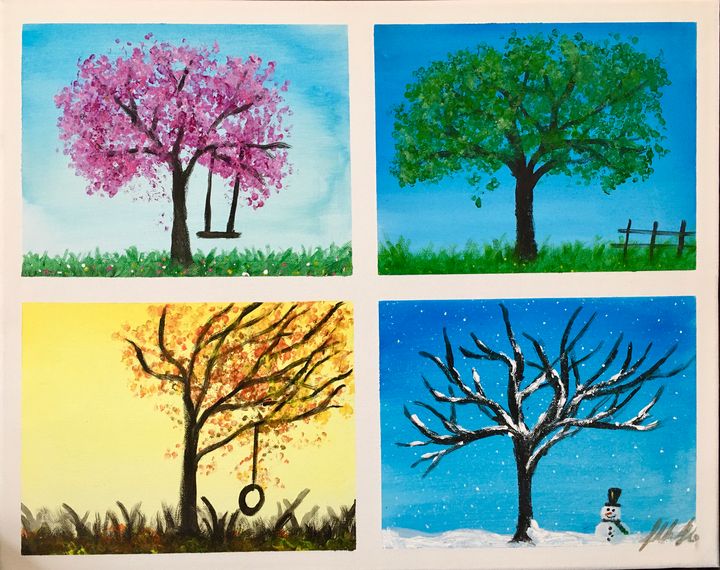This image is a traditional watercolor painting divided into four sections, each representing a season as seen through a window-like frame. The top left panel depicts spring, showcasing a tree with vibrant pink flowers and a swing hanging from its right branch. The sky is a bright blue, and the grass beneath is lush and green. Moving to the top right panel, summer is portrayed with the same tree now fully covered in green leaves. The background features a slightly darker blue sky, green grass, and a black fence to the right of the tree. The bottom left panel illustrates fall. The tree’s leaves have turned shades of orange, red, and yellow, and a tire swing dangles from a branch. The sky is a golden yellow, and the grass is dark, almost black. Finally, the bottom right panel represents winter, where the tree stands bare with snow covering its branches and the ground. The sky is a cold blue with white speckles, resembling falling snow. A small snowman, complete with a black hat, scarf, and buttons, stands under the tree. The artist’s signature is visible in the bottom right corner of this panel.